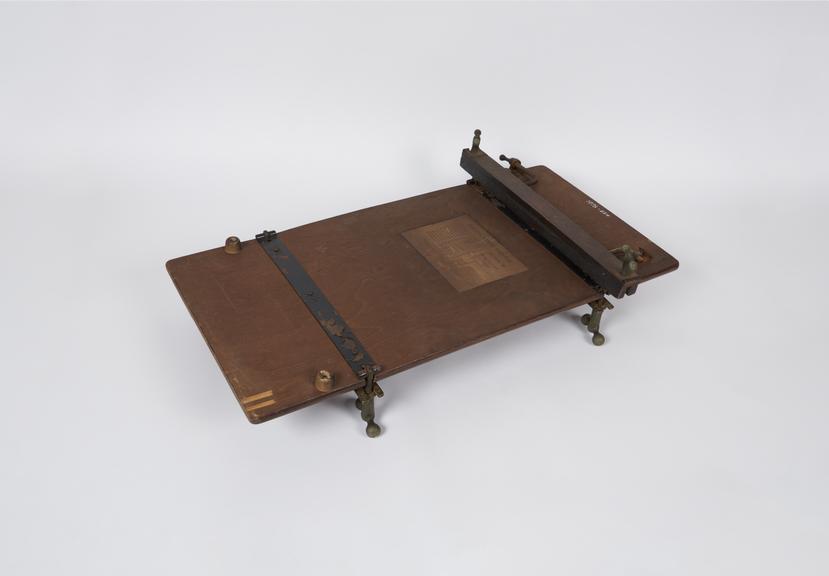This professional photograph showcases an antique, brown wooden device set against a white to very slight gray toned background. The object, which appears to be 50 to 100 years old, has a rectangular shape, possibly the size of a laptop and a half, though its size cannot be precisely determined due to the lack of a comparative object. The device features four metal legs with ball feet that support the main structure. Metal bars are present on either side of the top, with one bar looking adjustable and potentially for precision functions like cutting or shredding paper. At the center, there is a lighter, aged rectangular label that seems to have had writing or typeset, but it is now illegible. Additional features include a brown square in the center and a couple of knobs on the left edge, suggesting it could have been used for tasks such as drawing or precision work, though its exact purpose remains unclear.